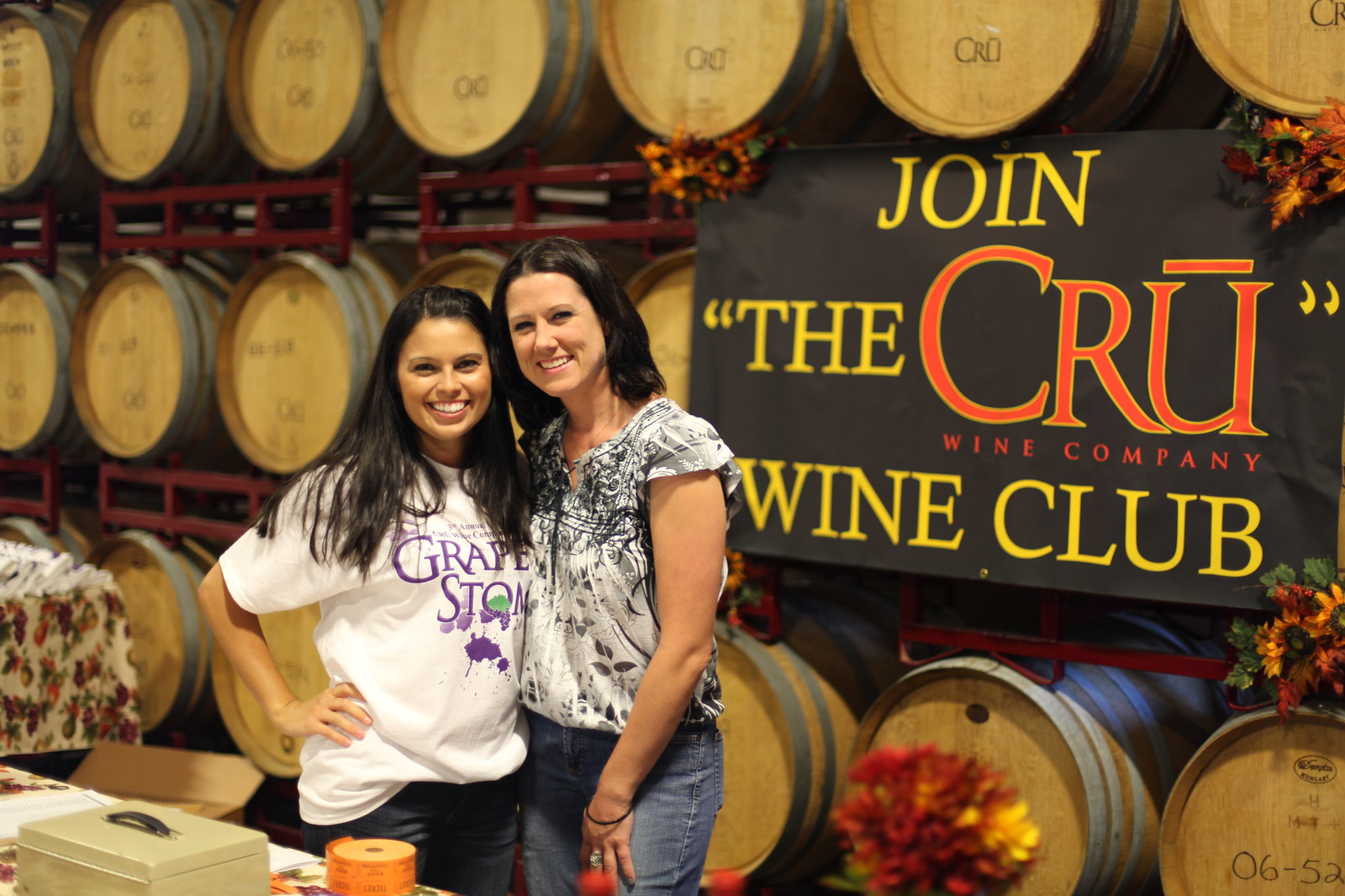In a well-lit indoor setting, this vibrant full-color photo features two attractive young women with dark hair posing together. Behind them, a large black sign with yellow and orange writing reads, "Join the CRU Wine Company, Wine Club," with "CRU" spelled C-R-U and accented with a line over the U. The backdrop showcases neatly stacked rows of oak barrels, presumably for wine aging, some of which display the number 0652. Additionally, a few bouquets of flowers are artistically placed near the barrels, adding to the ambiance. 

The taller woman on the left has darker hair and is dressed in jeans paired with a white shirt featuring a dark design. She has her hand on her hip. The shorter woman on the right, who has longer hair, is wearing a white t-shirt with purple text that says "Grape Stomp" alongside what appears to be grape splatter stains, accompanied by black pants. She has her hand resting on her thigh. Both women, smiling warmly, have their arms around each other's waists, exuding a sense of camaraderie. Near them, a table holds a cash box and perhaps tickets or flowery bags, complementing the inviting atmosphere of the scene.